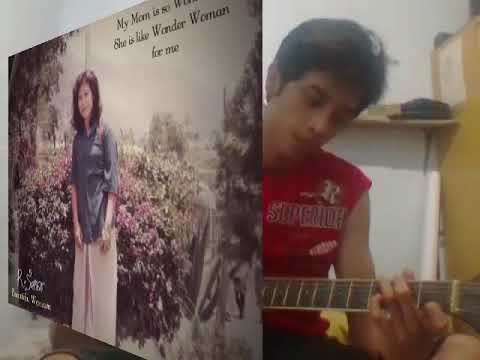In this image, there are two distinct panels side by side, centered within the frame and evenly spaced. On the left panel, there's an image of a woman standing in front of a vibrant flowering bush. The photo, which could be an album cover or a greeting card, features a partially visible inspirational message in black letters that reads, "My mom is so wonderful. She's like Wonder Woman for me." The background is predominantly white.

The right panel depicts a young boy or teenager with dark skin and dark hair, wearing a red sleeveless shirt. He is seated and strumming a guitar, with only the neck of the guitar and his hands visible as he looks down towards the instrument. Behind him, a white wall serves as the backdrop, along with a hint of a yellow or orange object to the right. The image appears to be a collection of personal photos, likely shared on social media, capturing a heartfelt and musical tribute.